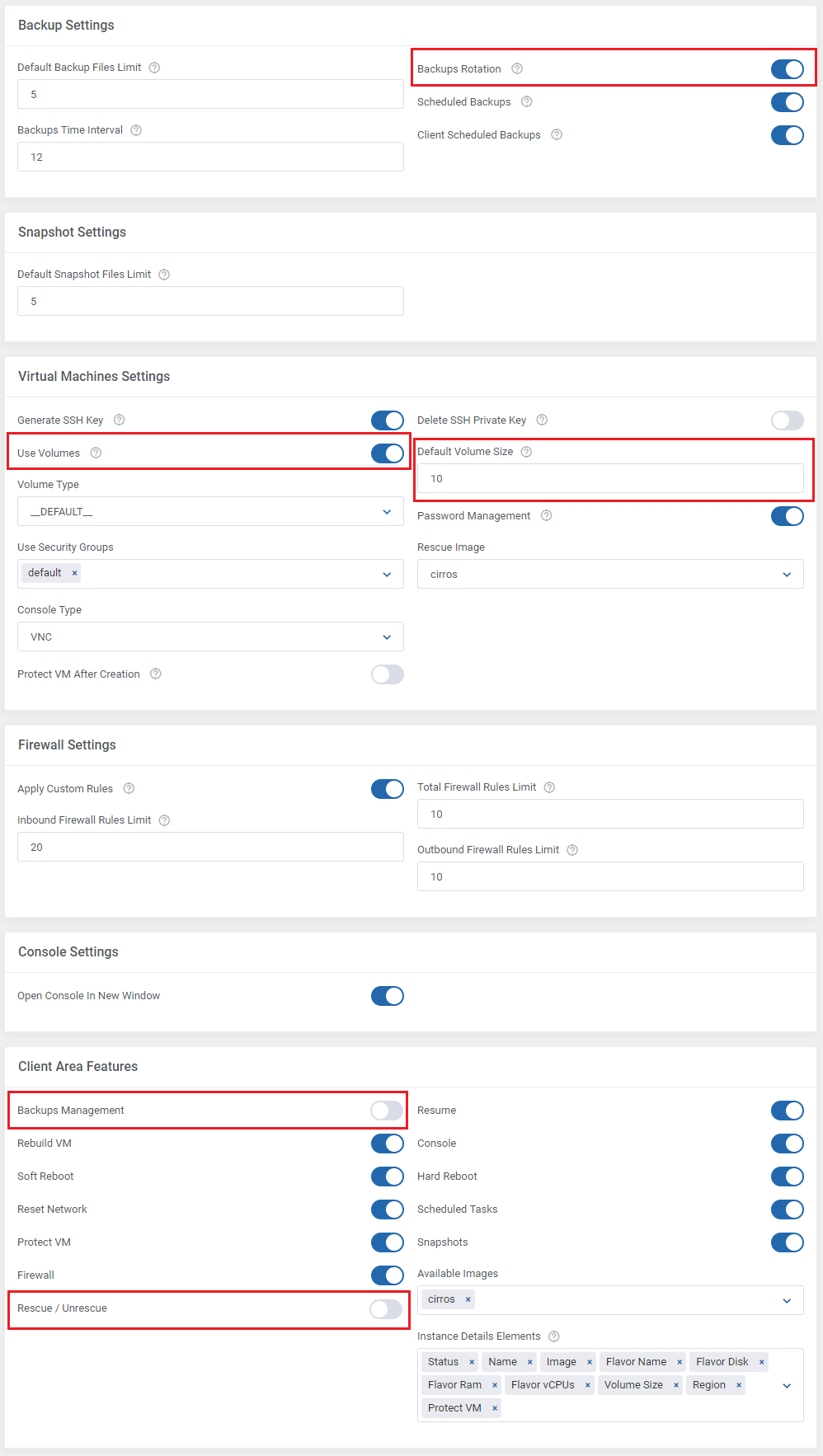The image depicts a screenshot of a settings interface, which is presented in a vertically aligned, light-colored rectangular frame. The interface appears to consist of multiple sections related to backup and system configuration.

The top section is labeled "Backup Settings" and provides details on various backup options. It shows that three features—"Backup Rotation," "Scheduled Backups," and "Client Scheduled Backups"—are enabled.

Below this, there is a "Snapshot Settings" section. It mentions "Default Snapshot," followed by an unreadable phrase, and includes a fillable input box.

The next section is "Virtual Machine Settings," which presents several columns of data in very small print, making the details hard to read.

Following this, "Firewall Settings" are shown, succeeded by "Console Settings."

At the bottom of the image, the final section is titled "Client Area Features."

Several elements within these sections are highlighted in red. In the "Backup Settings" section, "Backup Rotation" is emphasized. Additionally, in the "Snapshot Settings" section, a line involving "default" is marked in red, though the full text is unclear. Further, in the image, "User Volumes" and "Backups Management" are highlighted in red, and the words "Rescue / Unrescue" are circled with a red border.